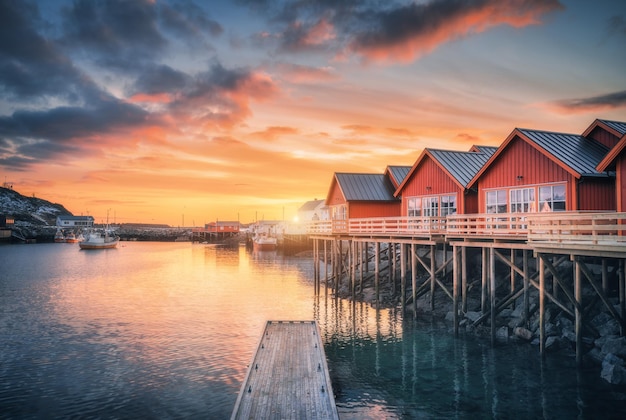The image captures a picturesque coastal scene during sunset. The sky is adorned with a blend of orange, pink, and gray clouds, casting a warm, colorful glow across the horizon. The sun, partially hidden, illuminates the sky and reflects beautifully on the tranquil water below. On the left side of the image, there is a hill and a mixture of dark water and sky in the lower and upper corners. In the center, a main pier with a simple rail extends forward, composed of vertical wooden planks. To the right, a rocky slope leads down to numerous wooden poles supporting several stilt houses. These distinctive houses feature vertical red slats, three lower windows, and dark gray triangular roofs. Behind them, additional buildings in white and red add to the charming coastal architecture. Some of these structures, also perched above the water, display the ingenuity of their design. The entire scene is bathed in the soft light of the setting sun, highlighting the serene interplay of natural and man-made elements.